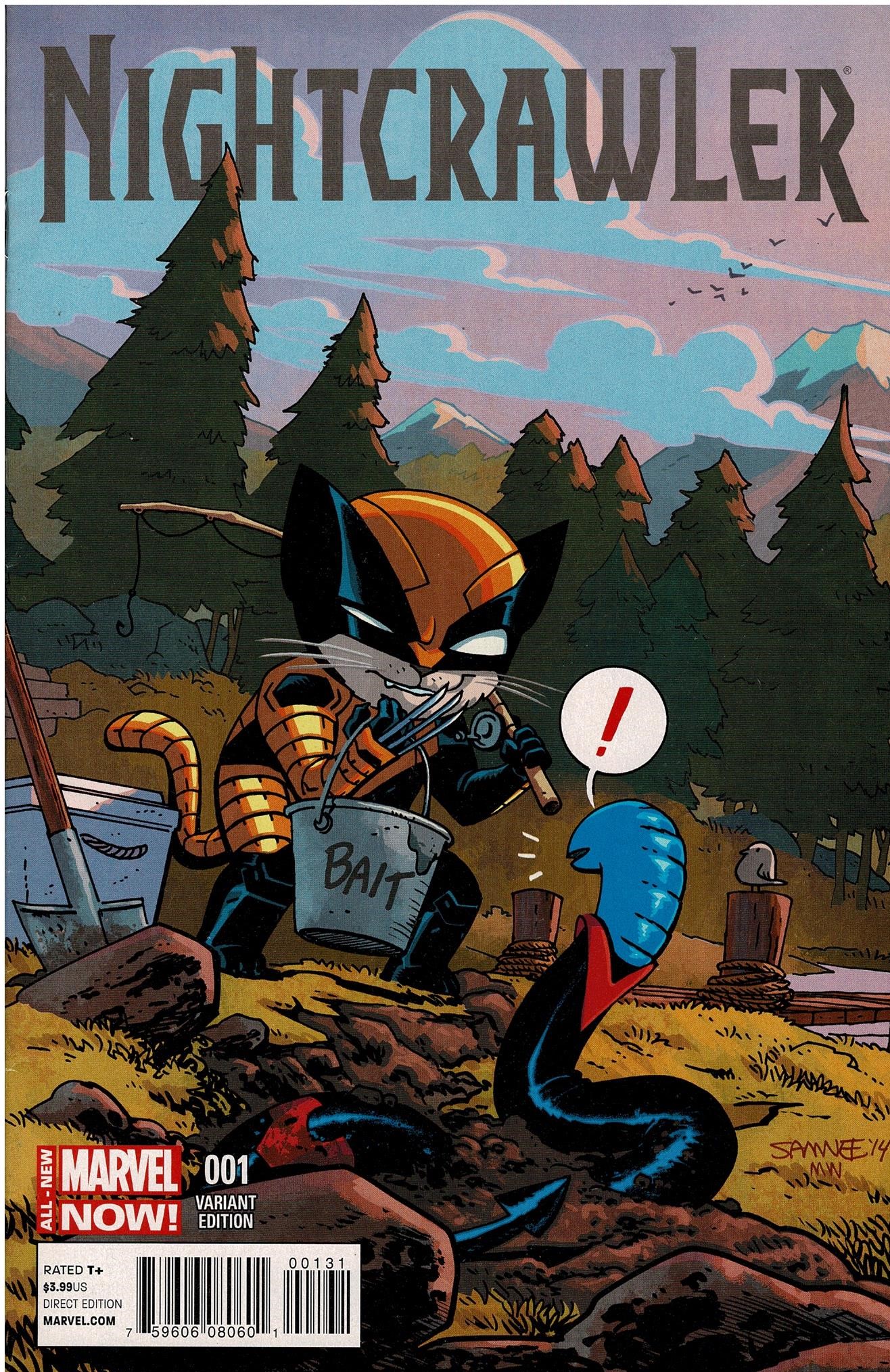The image is the cover of a Marvel comic book titled "Nightcrawler", featuring a playful and childlike illustration. Across the top of the cover, the text "Nightcrawler" appears in bold black letters against a backdrop of blue clouds. Centered in the image is a chibi-style Wolverine, characterized by a disproportionately large head, cat whiskers, a tail, and his iconic yellow and brown costume with long ears. Wolverine is crouching and holding a bait bucket labeled "Bait" with his claws extended. In the scene, dark-colored pine trees rise tall behind him and distant, snow-capped mountains peer above the horizon. Birds can be seen flying through the cloudy sky, adding to the whimsical outdoor setting. A large, blue worm with black and red accents—resembling Nightcrawler—is shown with an exclamation mark in a speech bubble above his head, indicating surprise or alarm. This worm is suggestively Nightcrawler transformed. A red label in the lower-left corner identifies the comic as a "Marvel Now! 001 Variant Edition." The setting appears to be near a dock and pond, reinforcing the fishing theme.